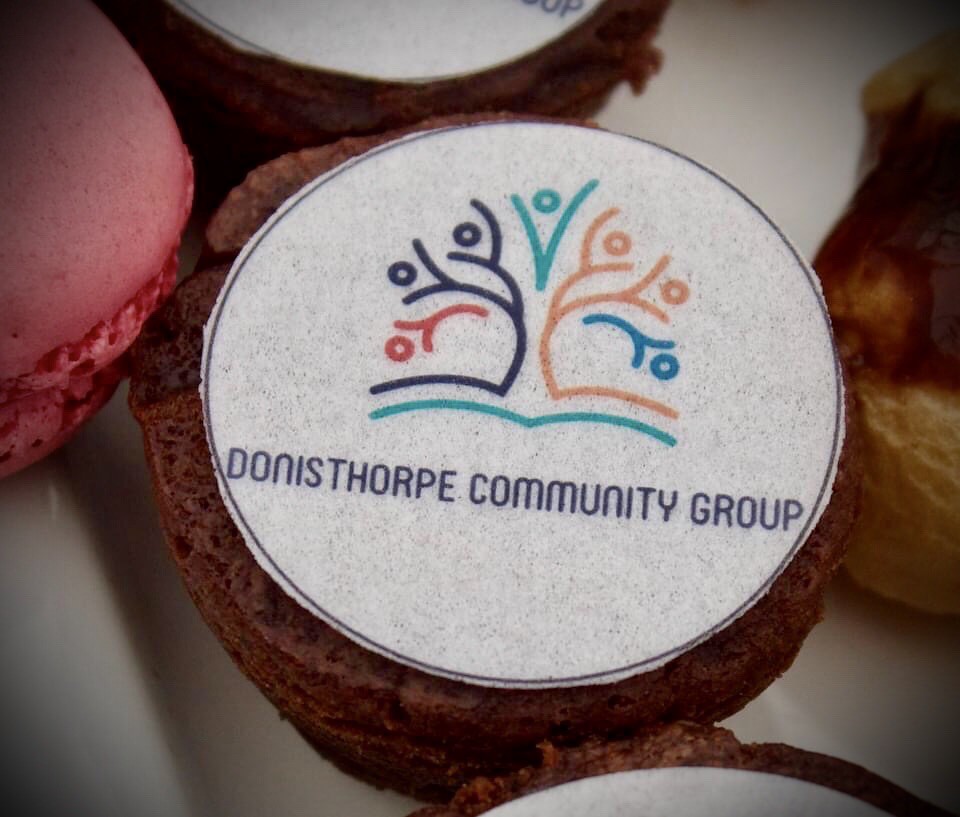The image showcases a variety of colorful macarons, including brown, pink, and light brown ones. Among them, one particular brown macaron stands out as it bears the logo of the Donisthorpe Community Group. This logo features a tree with branches shaped like human figures, rendered in vibrant colors including blue, orange, red, and cyan. Below the image of the tree, the text "Donisthorpe Community Group" is clearly visible. The detailed logo and text are printed on what appears to be a circular piece, possibly a coaster, placed atop the macaron, suggesting that the community group might be celebrating an event or occasion.